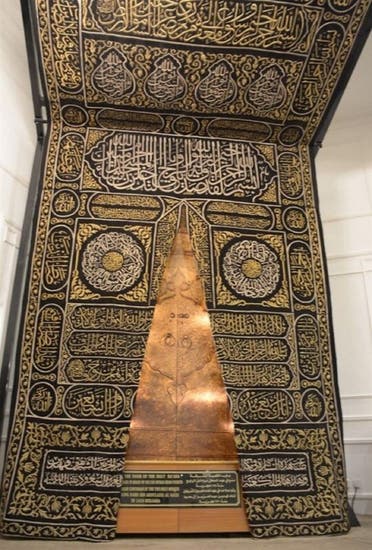The image depicts a close-up of a light brown, cone-shaped statue or artifact set against a gold-embellished tapestry that extends across the wall and ceiling of a textured white room. The statue, reminiscent of a trophy or ancient artifact, is detailed with intricate designs and features a plaque at its base with writing possibly in English and Arabic, though the text is too small to discern clearly. The tapestry behind the statue is richly detailed with gold, black, and some brown, showcasing various shapes like circles, ovals, and trapezoids, accompanied by what seems to be embroidery that may include Arabic calligraphy. The floor under the statue is a matching light brown, completing the room's aesthetically cohesive ambiance.